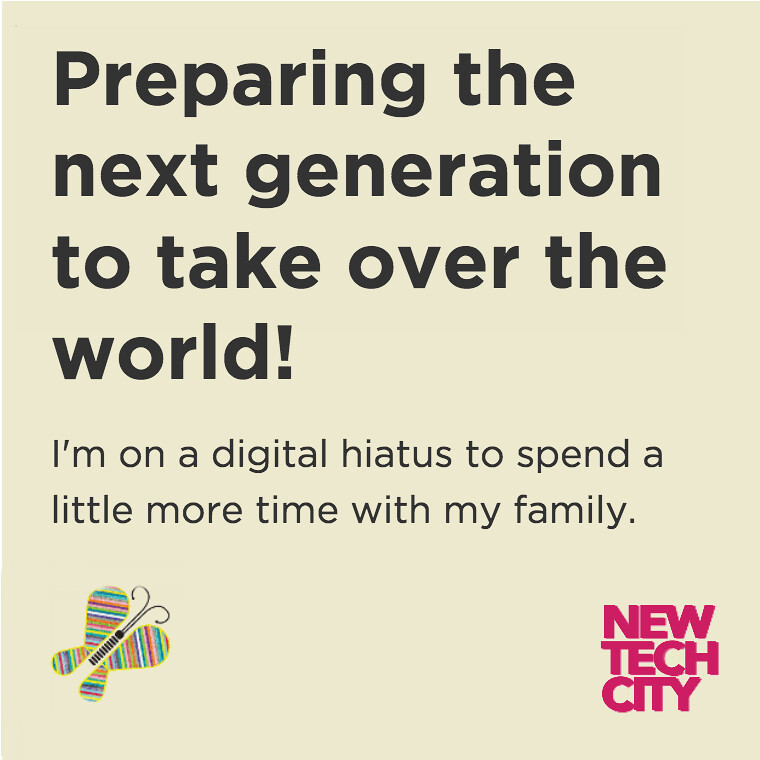The advertisement for New Tech City features a prominent title at the top in bold black text: "Preparing the Next Generation to Take Over the World!" Below this, in smaller black text, it states, "I'm on a digital hiatus to spend a little more time with my family." The background is a solid beige or creamy color. On the bottom left corner of the ad, there is an intriguing butterfly with wings outlined in yellow and filled with a vibrant mix of colors including blue, lighter blue, pink, orange, purple, green, and white. The butterfly has a black body with very long antennae and appears to be constructed from a spring for the caterpillar-like part and a circle for the head. On the bottom right corner, the logo for New Tech City is displayed in bold red block capitals.